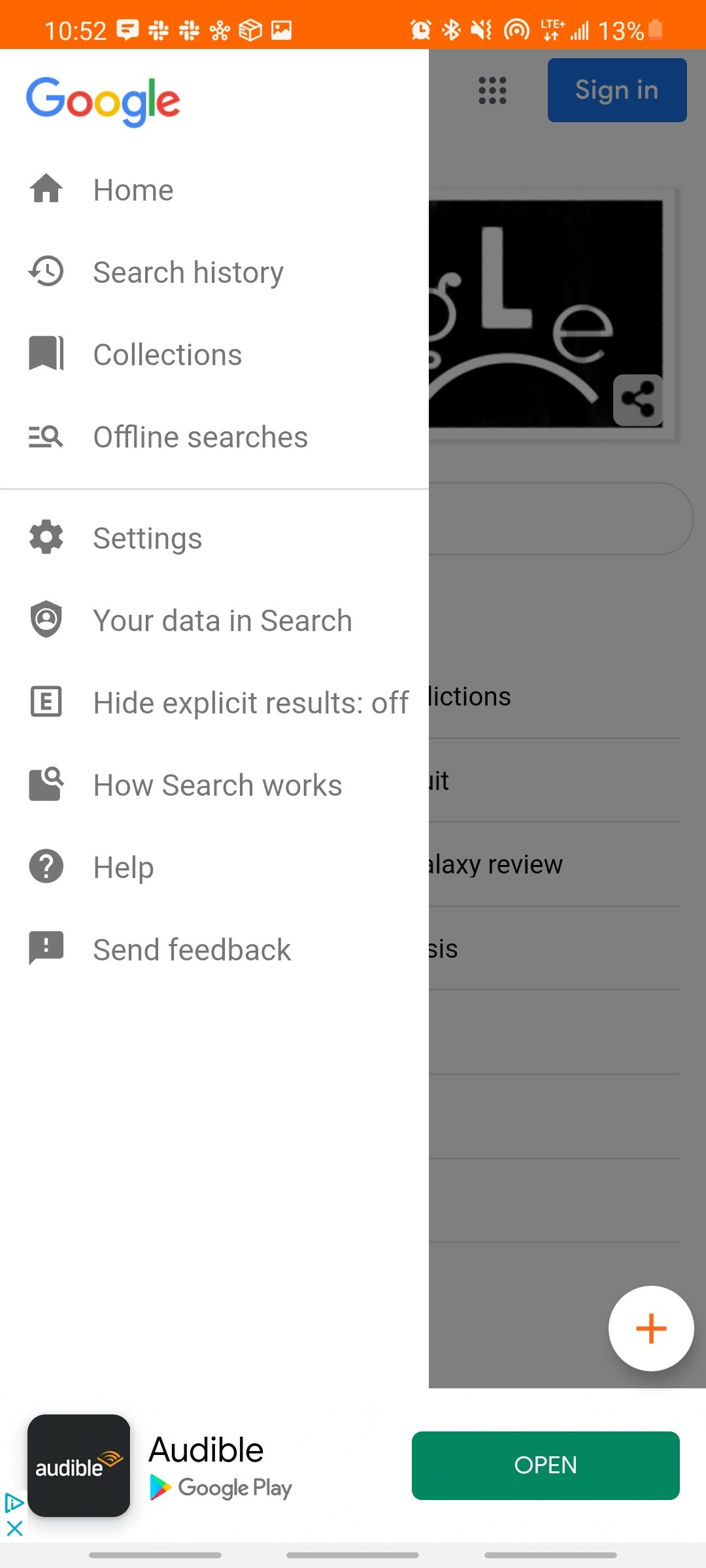In this image, the primary background is white. At the top of the image, there is an orange rectangular box displaying the number "1052" alongside an indicator showing the battery at 13%. Below this, the familiar Google logo appears in its traditional blue, red, yellow, and green colors. 

Underneath the logo, there are several options listed: "Home," "Search history," "Collections," and "Offline searches." Below that is a dividing line, followed by additional options: "Settings," "Your data in search," "Hide explicit results," "How search works," "Help," and "Send feedback."

At the very bottom left, a black square contains the Audible logo, accented with a gold element in one corner. The word "Audible" is present alongside a button labelled “Google Play,” which features a small triangle in blue, red, and yellow. Adjacent to this, further left, there are small icons: a tiny blue triangle and a blue X.

On the right side of the image, framed against a gray background, are nine dots arranged in a square formation and a blue "Sign in" button. The image also features a black box with the letters "GL" and an "E," accompanied by a curved line below them. In the bottom right corner, there's a small gray square with a sideways "V." 

Towards the bottom, black text is visible, alongside a white circle enclosing a red cross (or plus sign). Finally, a green button labeled "Open" is situated at the bottom of the image.